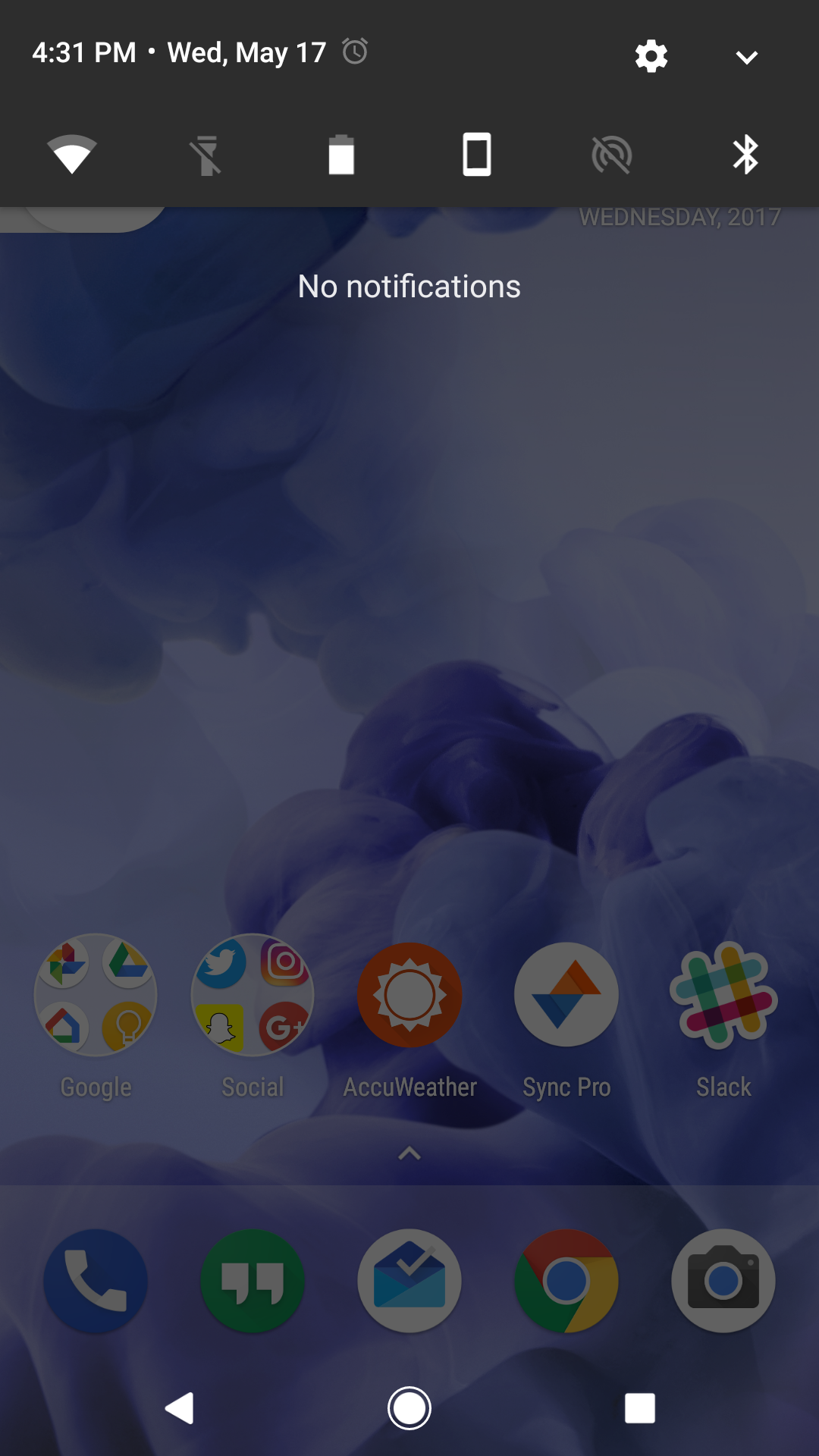The image captures a smartphone screen with a prominent grey border at the top. Displayed on the upper left corner of the screen is the time, 14:31 PM, and the date, Wednesday, May 17th. Adjacent to the date is a dimmed alarm clock icon, symbolizing an inactive alarm. To the far right, a small cogwheel icon indicates access to settings. Below this section, there is a row of status icons: a Wi-Fi signal, a disabled torch icon, a battery indicator showing the battery is mostly charged, a smartphone icon, two circles with a line through them, and a Bluetooth icon.

The central background of the screen resembles a cloudy blue-white chemical mixture or cloud formation. In white lettering at the top center of the display, it clearly states "No notifications." Near the bottom of the screen, various app icons are arranged, including Google, Social, AccuWeather, Sync Pro, and Slack.

At the very base of the phone, there is another set of icons: a blue icon featuring a phone, a green circle with two speech marks, a white circle with an envelope, the Google Chrome circle, and a grey circle with a camera in the center.